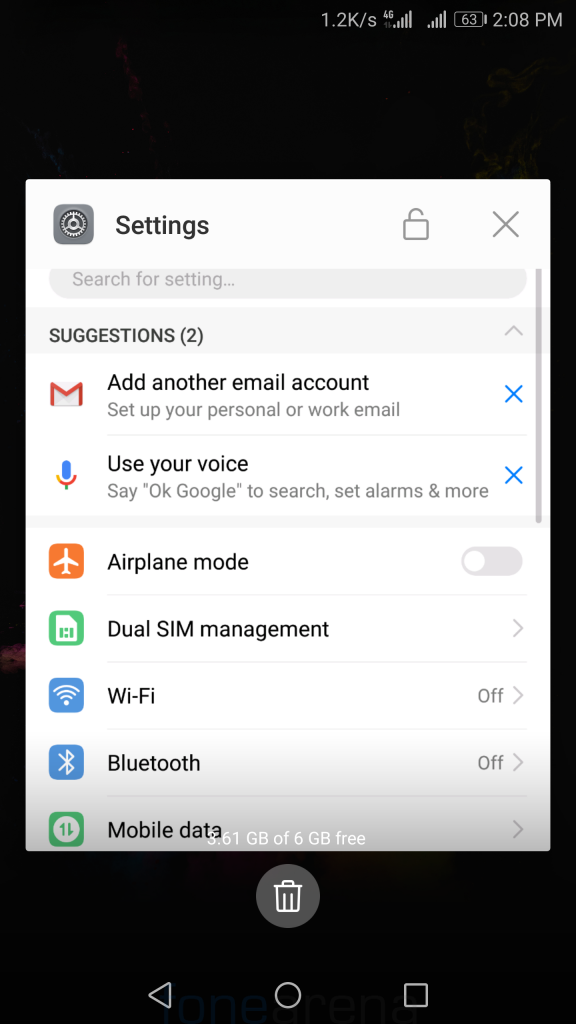### Detailed Caption for a Website Image:

The image is categorized under 'Websites' and showcases a smartphone with a black screen. The time displayed on the phone is 2:08 PM, and the battery level is at 63%. On the screen, there is a prominent white box labeled 'Settings' with a gear icon, indicating it is the settings menu. 

This menu includes a search bar at the top, which reads "Search for settings," followed by a section titled "Suggestions." The first suggestion, accompanied by an email envelope icon, is to "Add another email account," which prompts the user to set up their personal or work email. This suggestion can be dismissed with an X button or hidden entirely.

The second suggestion, marked by a microphone icon, is "Use your voice." It advises saying "OK Google" to perform various tasks such as searching the web and setting alarms.

Below the suggestions, key settings options are listed:
- **Airplane Mode**: Represented by an airplane icon.
- **Dual SIM Management**.
- **Wi-Fi**.
- **Bluetooth**.
- **Mobile Data**.

Additionally, there is an X icon that allows users to close the Settings menu. The interface is user-friendly, integrating both graphical icons and textual descriptions to help users navigate and manage their device settings effectively.